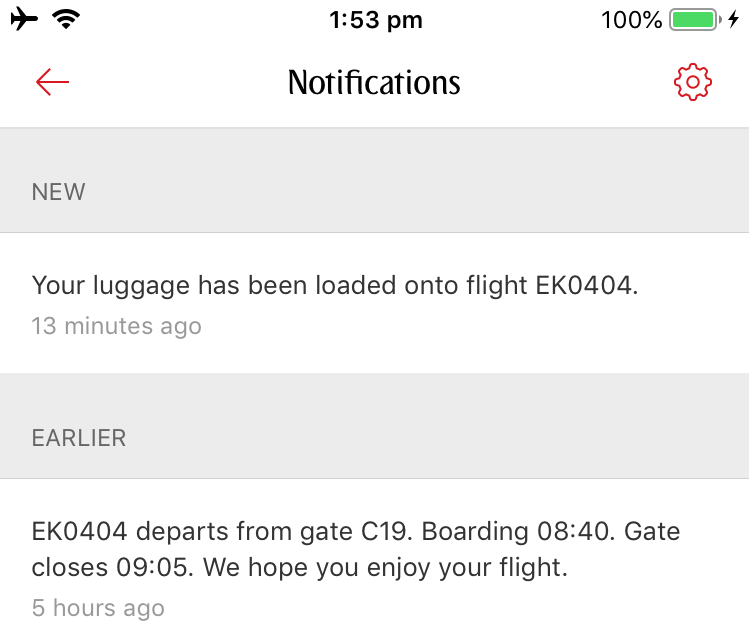The image depicts a notification screen on a white background. In the top left corner, a black airplane icon is seen flying to the right, accompanied by a Wi-Fi icon. At the top center, the time is displayed as 1:53 PM. In the top right corner, it shows "100%" next to a fully green battery icon with a lightning bolt, indicating that the device is charging.

Below these, there is a red arrow pointing to the left, followed by the word "Notifications" in black text. To its right, there is a red cogwheel icon. Underneath this header, the notification section begins.

A gray box labeled "New" is followed by a white box containing the message: "Your luggage has been loaded onto flight EK0404 13 minutes ago." Another gray box below states: "Earlier EK0404 departs from gate C19. Boarding 8:40 AM, gate closes at 9:05 AM. We hope you enjoy your flight."